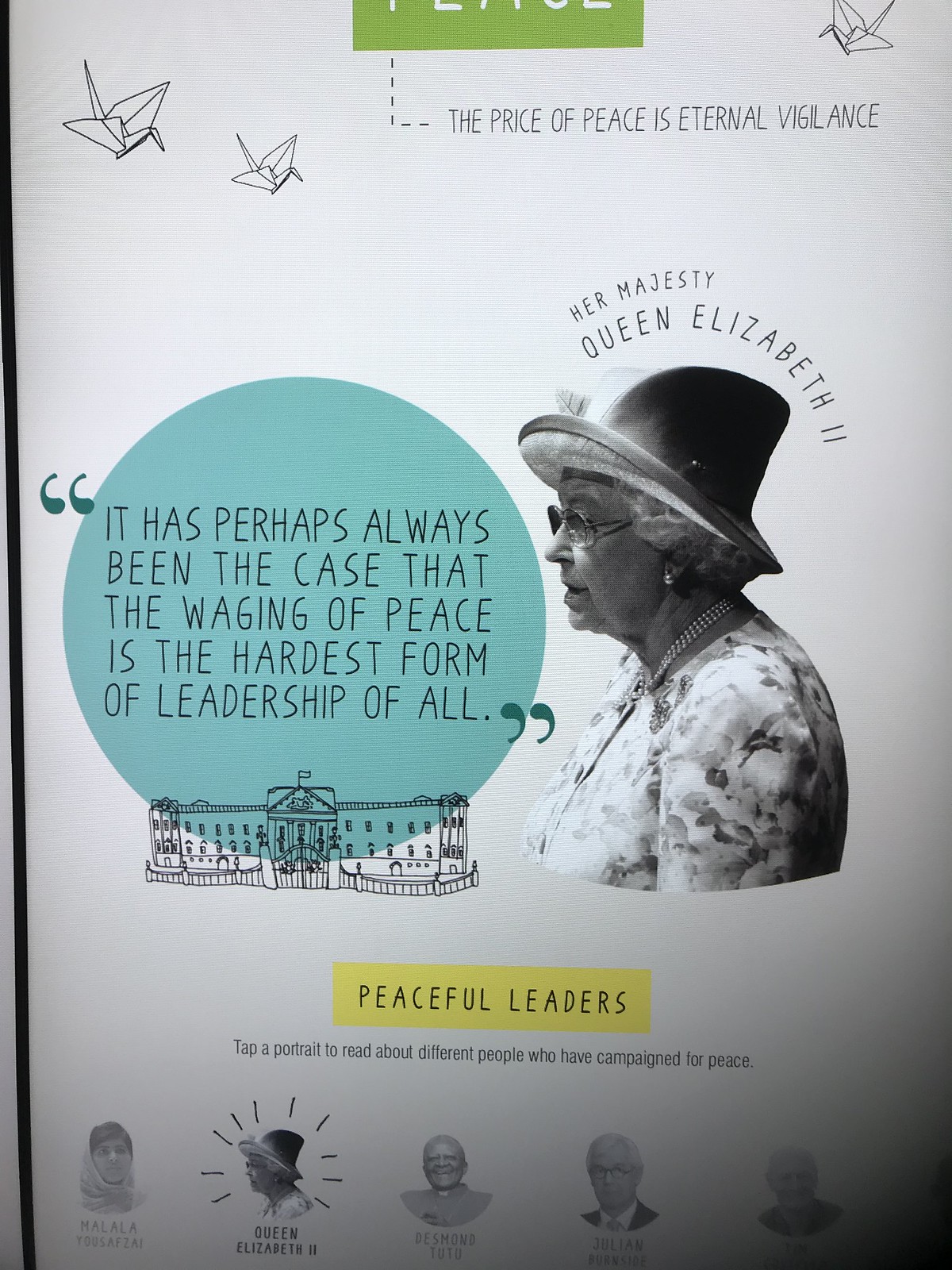This detailed image features a montage with various cutouts centered around a black-and-white photo of Queen Elizabeth II, labeled "Her Majesty Queen Elizabeth II." In the image, the Queen is depicted wearing a hat, a white dress, a jeweled necklace, and glasses. Above the portrait, there is a green sign with white letters, though the text is not readable. Beneath the Queen's photo is a blue balloon with quotation marks containing the text, "It has perhaps always been the case that the waging of peace is the hardest form of leadership of all."

To the left of the Queen's image is a rudimentary drawing of Buckingham Palace. Below this, in a yellow box, it reads "Peaceful Leaders." Underneath, the caption lists several figures recognized for their peaceful leadership, including Malala Yousafzai, Queen Elizabeth II, Desmond Tutu, and Julian Assange, though some details are faded and another leader's name is not fully visible. At the bottom of the page, additional leaders are mentioned, but specific individuals like Donald Trump are not depicted. Below the Queen’s image, in plain script, it states, "The Prince of Peace is Eternal Vigilance," reinforcing the overall theme of peace and leadership.